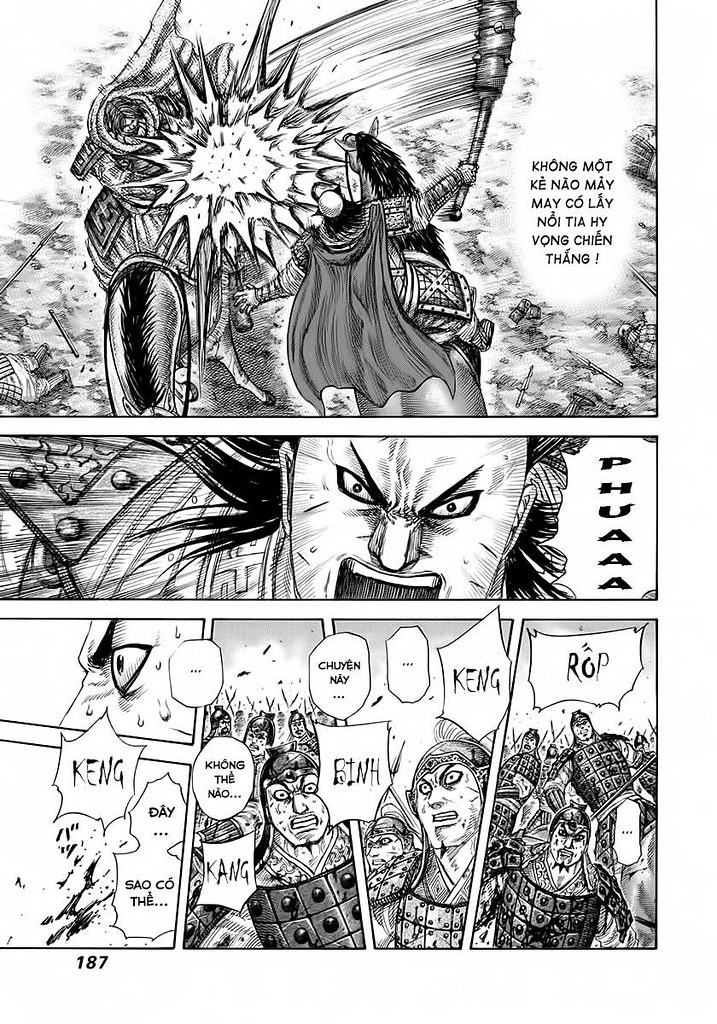The image depicts a dynamic comic book page in black and white, displayed on a white surface. The page is divided into several panels, each showcasing a series of intense and dramatic scenes. At the top, there is a depiction of two armored warriors on horses charging towards each other from opposite directions. The warrior on the right is swinging a massive war club, creating an impactful strike against his opponent. 

In the center panel, a close-up captures the fierce expression of one warrior, his face contorted in a fearsome yell. Adjacent to this, another close-up panel shows a different warrior, wide-eyed and sweating, conveying a sense of intense anxiety. Following this, there's a smaller panel displaying a splatter of blood, indicative of the violent encounter.

Toward the bottom of the page, several panels feature different soldiers. The first group of soldiers appears alarmed and fearful, their expressions conveying the chaos of battle. The subsequent panels show these soldiers increasingly bloodied and more visibly agitated, their nervousness escalating with each scene. The comic book's language is unreadable, adding an element of mystery to the narrative, and the entire composition, with its detailed shading, firmly places it in a dramatic gray-scale aesthetic reminiscent of war-themed comics, possibly from the Vietnam era.